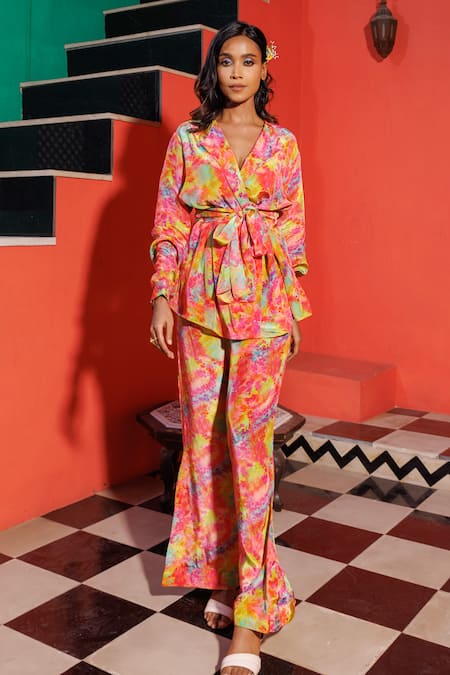In this striking image, a tall, slender woman, who appears to be a model, stands poised in a vibrantly colorful, matching ensemble. Her outfit, featuring a tie-dye pattern predominantly in pink, splashed with hues of blue and yellow, consists of flared pants and a long-sleeve wrap top tied at the waist with a sash. She complements her look with white sandals that wrap around her feet. Her hair, adorned with floral decorations, is neatly parted with one side tucked behind her ear, accentuating her tan skin and the light blue glittery eyeshadow that graces her eyes. She stands on a black and white checkered floor, with a graphic and vividly colored background enhancing the bold aesthetic. The backdrop includes a red wall, black stairs, an orange accent wall, a small table, and a light fixture, lending a dynamic and somewhat eclectic atmosphere to the scene. The overall setting, possibly a staged backdrop, contrasts with her natural makeup look which features prominently blue eyeshadow and a subtle lip color, adding to her striking presence in the photograph.